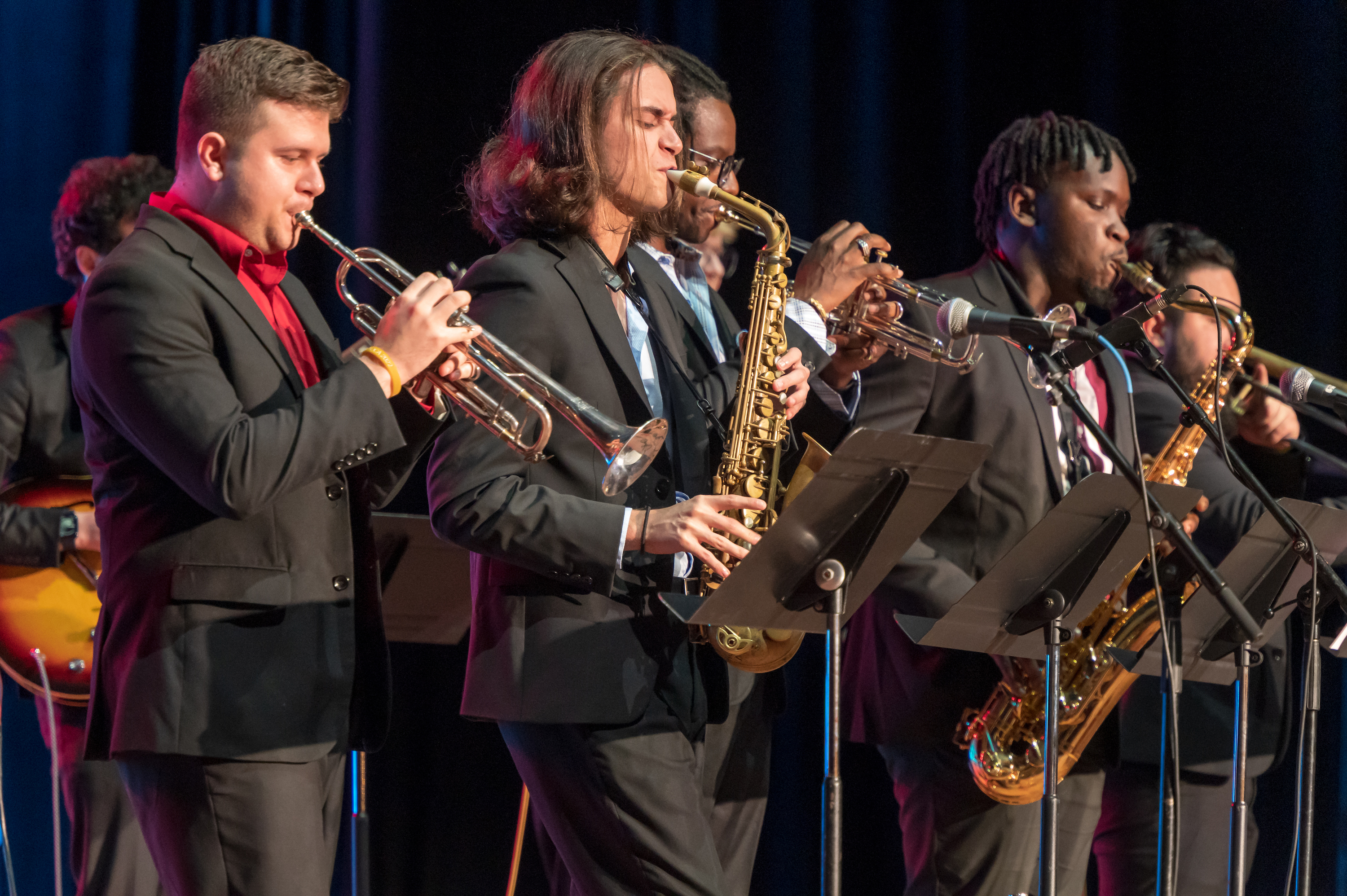This photograph captures a diverse group of male musicians performing on stage, illuminated by spotlights. They are all donning formal black suit jackets paired with different colored shirts underneath and charcoal gray pants. From left to right, the performers are organized as follows: 

- A light-skinned man with short brown hair in a red shirt, playing a silver trumpet.
- A man with long brown hair in a blue shirt, standing behind a black music sheet holder and playing a golden saxophone.
- A dark-skinned man with dark hair in a blue shirt, partially obscured, playing a trumpet.
- A dark-skinned man with black dreadlocks in a white and red striped shirt, playing a saxophone with a music stand in front of him.
- Another mostly obscured person, possibly playing an instrument, is also visible to the right.

A guitarist can be seen behind the front row of musicians, adding to the ensemble's rich sound. The lineup faces towards the right side of the image, with a black microphone stand leaned in from the right. The background features a dark blue curtain that fades to black towards the right side, further highlighting the performers.